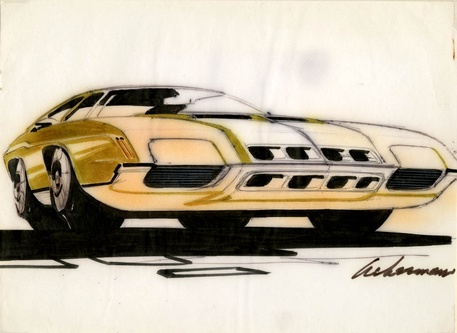This image displays a meticulously crafted drawing on an aged, yellowed piece of paper, signifying the passage of time. The paper, now subtly faded, bears an artist's signature in the bottom right corner, although the signature is difficult to decipher and appears to read something like "Ash Demon." The focal point of the artwork is a sports car, presented in a cartoonish, stylized manner rather than a realistic depiction. The car is adorned with shades of white and gold. On the left side of the drawing, the tires are disproportionately large, almost reminiscent of monster truck tires, creating a striking contrast with the more conventionally sized tires on the right side, of which only the bottoms are visible. The unique perspective and creative exaggeration highlight the artist's imaginative approach to the subject matter.